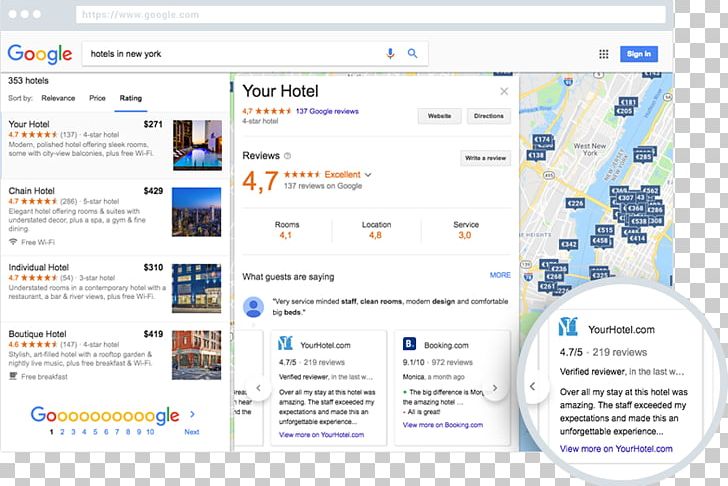In this image, we see a Google search results page displaying a query for "hotels in New York." On the screen, the search bar containing the query is prominently featured at the top, accompanied by the microphone icon and the search button to its right. Below the search bar, the results indicate that there are 353 hotels listed. 

One highlighted option is a hotel rated 4.7 stars based on 137 reviews, with a price of $271. The search results also mention a chain hotel priced at $429 with a 4.7-star rating and a boutique hotel priced at $419 with a 4.6-star rating. Additional details about the hotel rooms are provided, including a 4.1 rating for the rooms themselves, a 4.8 rating for location, and a 3.0 rating for service.

The description also includes feedback from guests, noting that the staff is very service-minded, the rooms are clean with modern design, and the beds are comfortable and large.